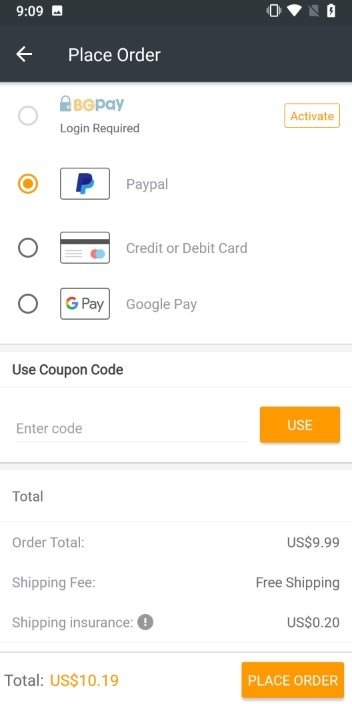A screenshot of an online order page is displayed. At the top, the time is indicated as 9:09, along with various status icons including a phone on vibrate, battery power, and internet connection signal. Below, a black rectangular banner with white text reads "Place Order," accompanied by a left-pointing arrow on the left side.

Further down the page, there is a "BG PAY" logo with a lock icon next to it, indicating a secure payment gateway. The section shows four payment option buttons, arranged in a column. The second option, highlighted in yellow, is PayPal. Other payment options include Credit/Debit with a card icon, Google Pay with its respective logo and text, and a button labeled "Activate" to the right side of this payment section.

An additional note beneath the BG PAY section reads "Login Required." A "Use Coupon Code" field appears next, with a box to enter the code and a button labeled "Use."

At the bottom, the order summary lists the total amount as $9.99 USD. A free shipping offer is noted, while the shipping insurance adds an extra $0.20 USD. The final amount displays as $10.19 USD. The page culminates with a prominent "Place Order" button, inviting users to finalize their purchase.